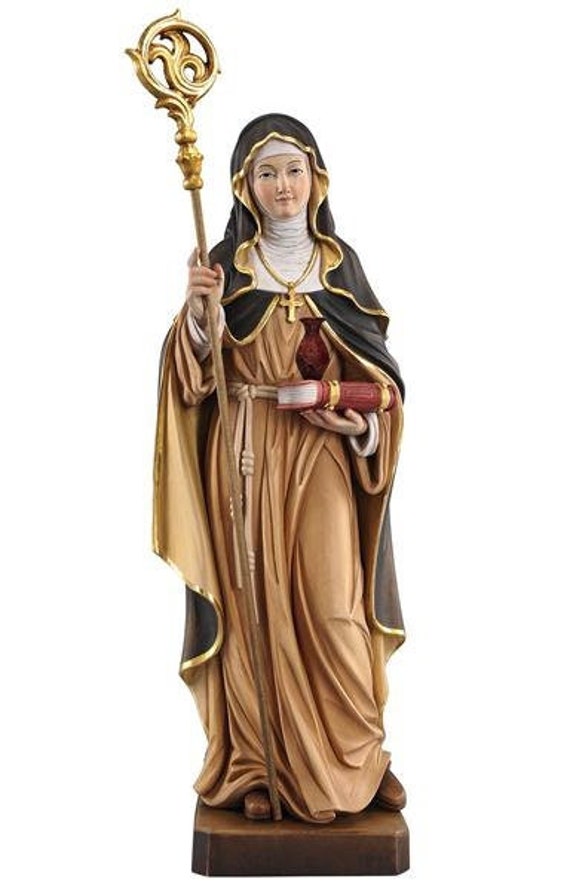The image depicts a highly detailed religious figurine made of either clay or ceramic, symbolizing Christian, perhaps Catholic, iconography. The female figure is adorned with a gold necklace that features a prominent cross in the center, highlighting its religious significance. She is garbed in a soft camel-colored robe, over which she wears a black cloak with a gold-rimmed hood. The inner lining of the cloak is also gold, creating a striking contrast. In her left hand, she grasps a gold staff with an intricate design at the top and a bronze base resting near her right foot. Her right hand holds a large red book with gold binding, atop which sits a red vase. The figurine stands on a brown base, and the overall scene is set against a clean white background with no accompanying text. The detailed craftsmanship, from her brown shoes to the intricate adornments and the serene expression on her white face, make this figure a captivating representation of devotional art.